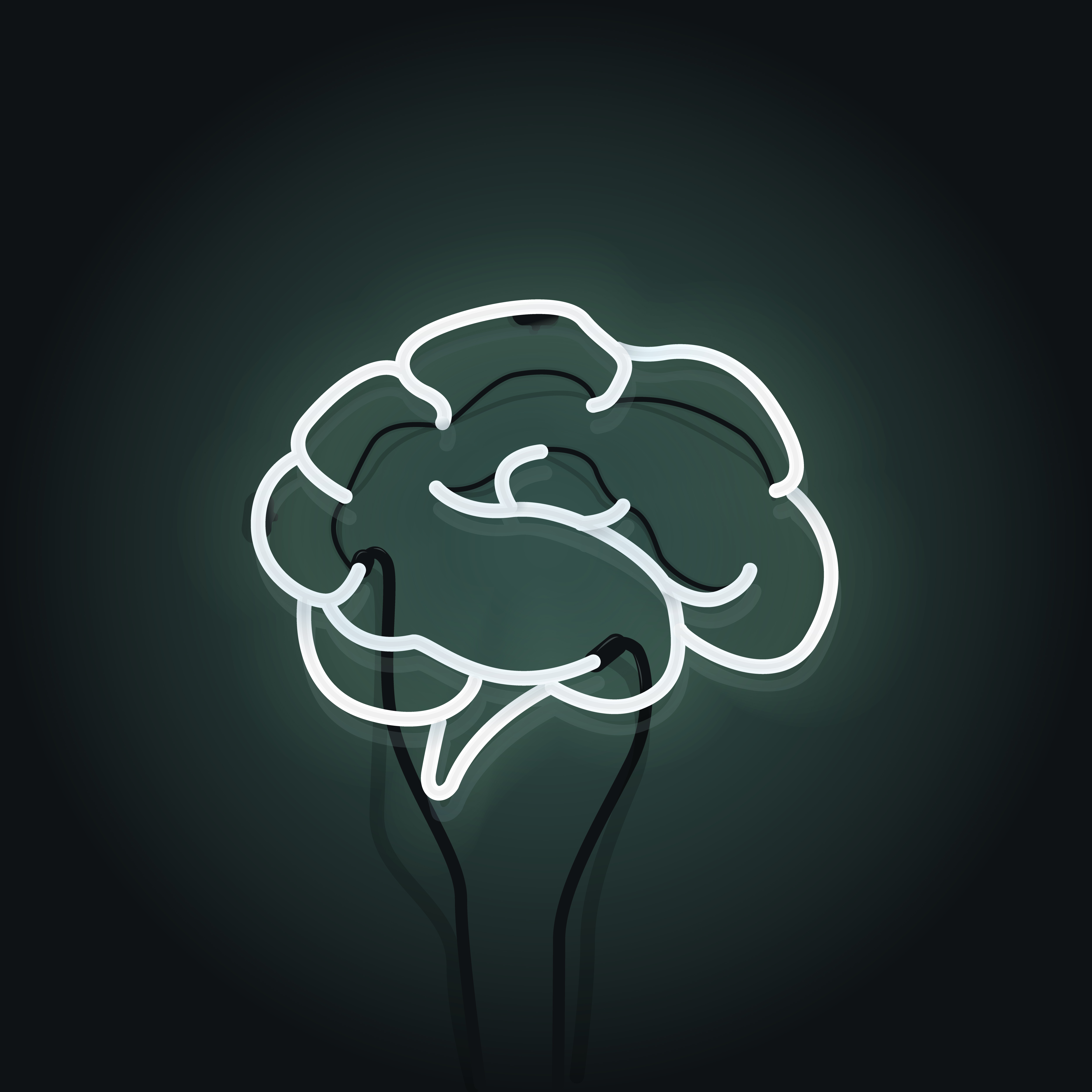In this image, a neon light sculpture emits an ethereal glow against a dark background, casting a mysterious ambiance. The sculpture seemingly represents a human head, outlined in black, with intricate white neon tubing delineating what appears to be a brain overlaying the head. Two black lines, likely electrical connectors, rise from the bottom, powering the neon lights that curve and intertwine to form the illuminated "brain." The backdrop features a circular gradient, transitioning from light gray in the center to a dark gray edge, enhancing the contrast and drawing the viewer's attention to the luminous artwork. The black-painted tubing emphasizes the visual impact of the glowing white lines, creating a compelling focal point in the dimly lit scene.